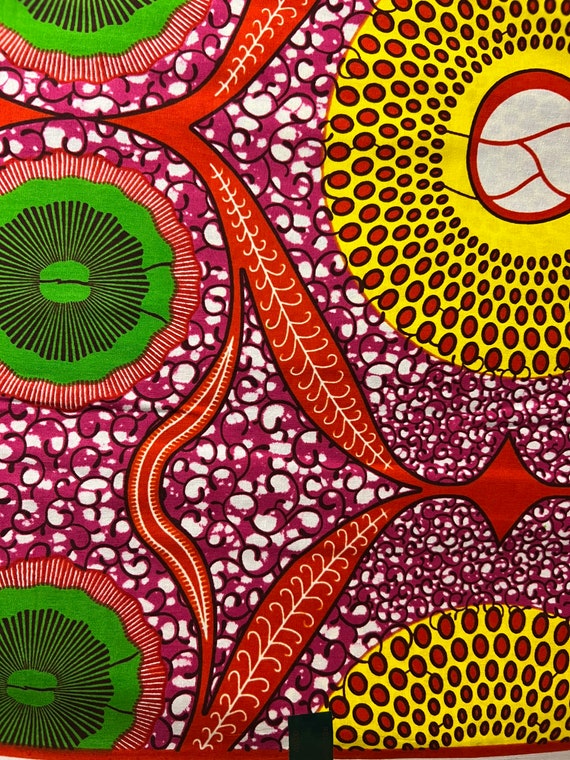This image features a highly detailed, colorful abstract design dominated by circular motifs and intricate patterns. On the left-hand side, three vertically aligned circles exhibit a repetitive pattern. Each circle has an outer red ring encircling red and white lines, a wavy-bordered inner green segment, and thin black lines radiating outward from the center. The background showcases a dynamic mix of white, pink, and purples adorned with black squiggly lines, evoking a kaleidoscopic effect. Prominent orange stripes, outlined in black with white zigzags within, run down the center of the piece. On the right-hand side, two large yellow circles with small red dots grow larger in a sequential pattern. Additional elements include floral and leaf designs with red, white, and green hues, contributing to the mosaic-like appearance reminiscent of intricate floor tiles.